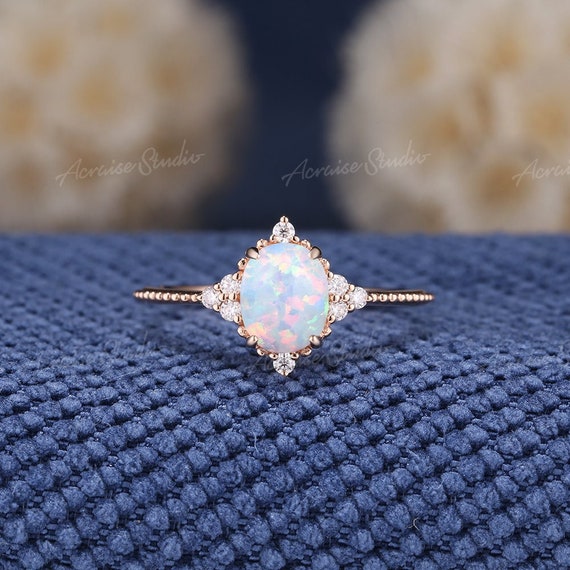This close-up photograph features an intricately designed ring placed on a dark indigo-blue, quilted cloth. The backdrop includes two blurred, white, puffy objects resembling bouquets of flowers, adding a sense of depth to the image. Dominating the top third of the photograph is a cursive watermark that reads "Arceis Studios," repeated three times in white. The centerpiece, a luxurious ring, stands out with its dark metal band adorned with small, evenly spaced white gems. At the heart of the ring is a striking, faceted gemstone that transitions in color from light blue to pink, encircled by a gold rim. Surrounding the central gem, three slightly larger stones are arranged in triangular formations on each side, complemented by additional gems at the top and bottom. Four darker metal prongs secure the main jewel, adding to the ring's elaborate design. The woven pattern of the indigo-blue cloth enhances the ring's prominence, making it the focal point of this elegant composition.